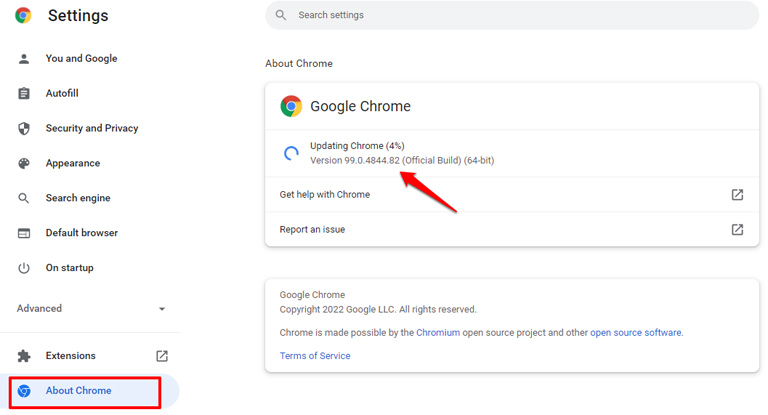This photo captures the "Settings" page in Google Chrome. At the top-left corner, there's a recognizable Google icon. To the right, the word "Settings" is prominently displayed in bold, black letters. Below this header, on the left-hand side, there is a vertical list of categories arranged in the following order: "You and Google" at the top, followed by "Autofill," "Security and Privacy," "Appearance," "Search Engine," "Default Browser," and lastly, "On Startup."

Further down, there's another category titled "Advanced," which features a drop-down menu. Underneath "Advanced," two more options are visible: "Extensions" and "About Chrome." The "About Chrome" section is highlighted with a red rectangle, indicating that it is currently selected. 

On the main pane of the page, the "About Chrome" section is displayed. At the top, there is a search bar labeled "Search settings." Below this, a prominent heading reads "About Chrome." Dominating the page is a large box titled "Google Chrome," featuring the Google logo beside the text. Beneath this, the message "Updating Chrome 4%" is shown, along with the version number and "Official Build 64-bit." Additionally, a red arrow has been edited into the image, pointing directly at the version number for emphasis.